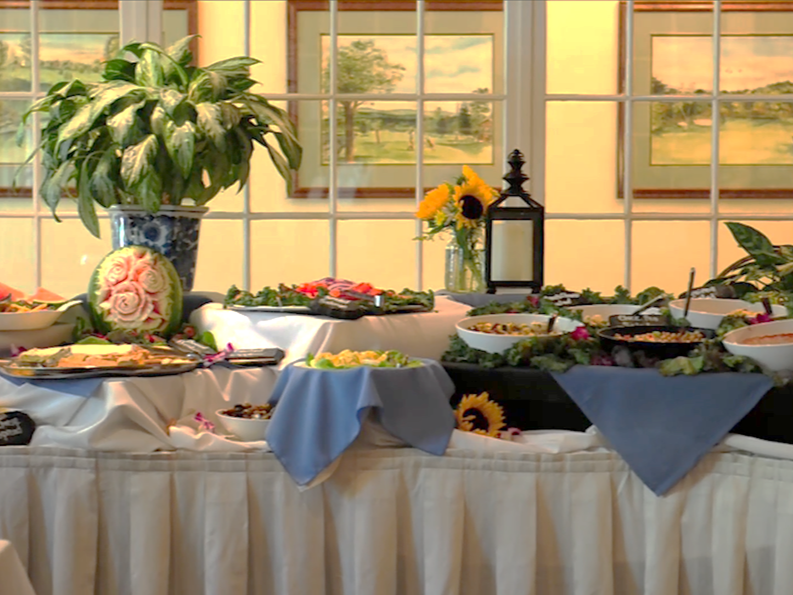The image depicts a sumptuous banquet table laid out on a three-tiered stand, draped in an immaculately pleated white tablecloth, with its lower fringe rippling elegantly. The table's clean and inviting appearance is enhanced by several royal blue linen napkins lining the platforms where bowls of vibrant cold salads, fruits, vegetables, and beans are arranged. Adding to the aesthetic appeal are delicate floral decorations, including a clear jar with sunflowers at the center and a Delft print planter with a bushy green plant in the back left corner. Behind the table, a multi-pane window with wooden white frames offers a view into a hallway adorned with three framed landscape paintings on a beige wall. The setting is softly illuminated by natural, low-key lighting, casting a warm and welcoming glow over the entire arrangement.